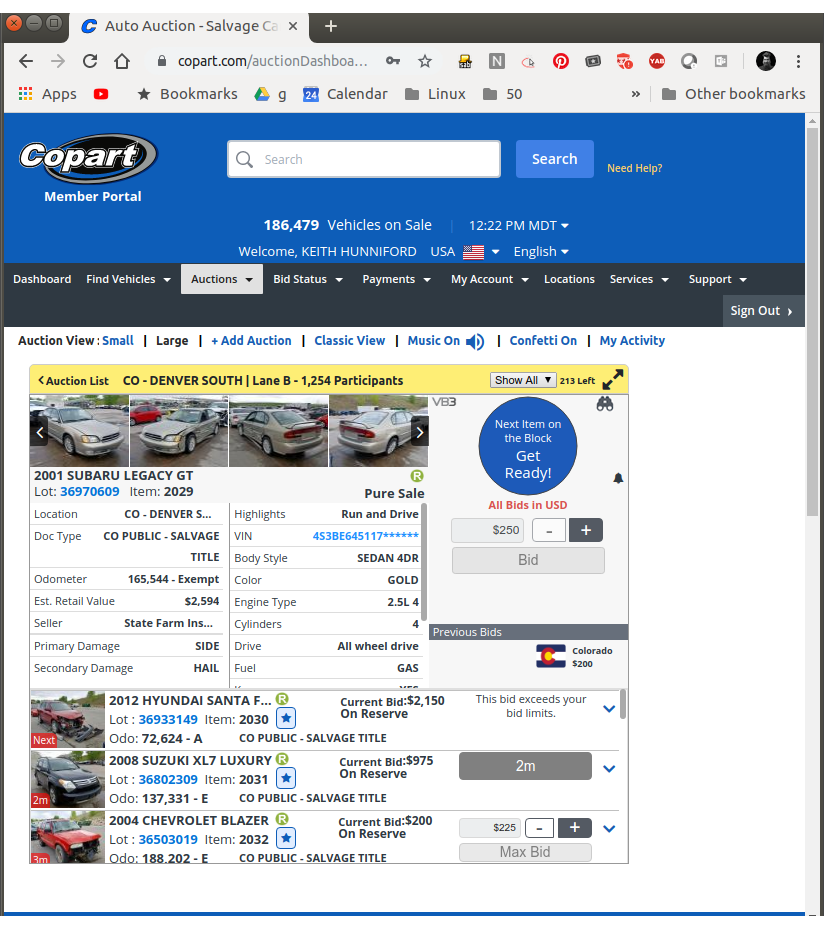This image captures the auction dashboard on the Copart website, visible through a browser. The URL "copart.com/auction-dashboard" is displayed in the address bar, indicating the specific section being viewed. The browser tab is labeled "Auto Auction - Salvage." The website presents an interface reminiscent of traditional search engines.

In the upper left corner of the webpage, within a blue top banner stretching across the screen, the Copart logo and the words "Member Portal" are prominently displayed. To the right of this section, there is a gap followed by a search bar and a search button.

Just below the search bar, a banner indicates that there are 187,479 vehicles available for sale. The current time displayed on the webpage is 12:22 p.m. MDT (Mountain Daylight Time).